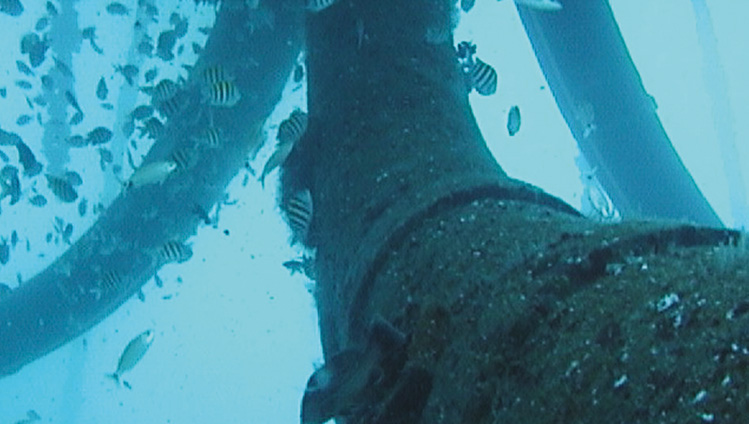This image depicts an underwater scene featuring three large, metal pipes, each approximately 15 inches in diameter, which are positioned horizontally and are curved within the frame. The pipes appear old and are densely covered in algae and fuzzy green moss, indicating they have been submerged for a significant period. The central, dark gray or brown pipe, which starts from the middle top of the image and extends down toward the lower right corner, dominates the scene. Flanking it are two other pipes in the background, each curving toward the sides of the image.

The water surrounding the pipes is a light, somewhat dingy blue, giving a foggy and hazy appearance. Teeming around these pipes is a large school of tropical fish. These fish exhibit distinctive tiger-striped patterns in black and either silver, white, or very pale yellow, with oval-shaped, wide bodies. Their vibrant, striped appearance contrasts with the muted tones of the pipes and the greenish algae. The fish seem to be attracted to the pipes, possibly due to the warmth or shelter they provide, and their presence adds dynamic life to the underwater setting, which could be part of an ocean environment or even an aquarium.